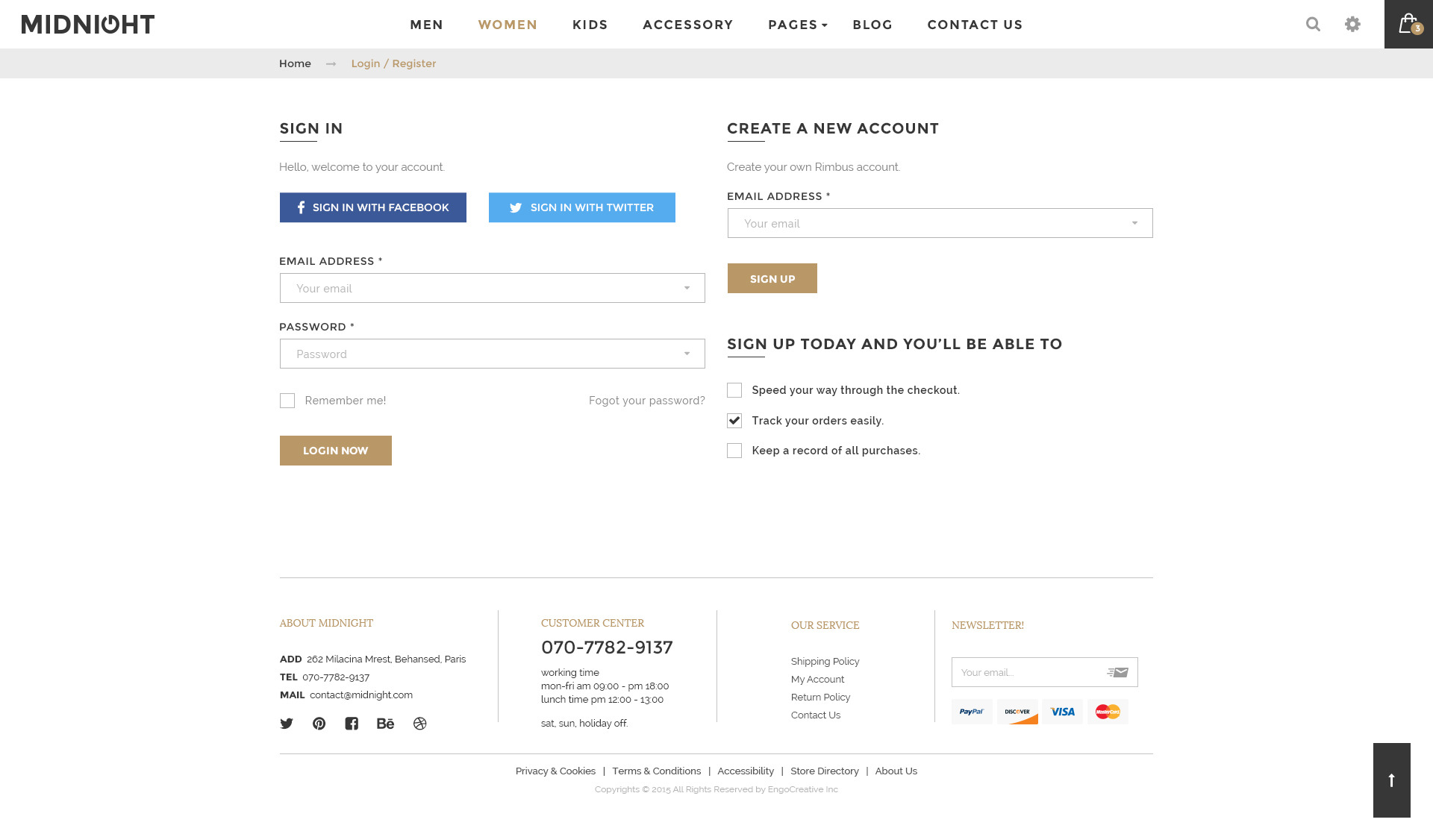The image depicts a webpage from a retail website called "Midnight," as indicated by the logo in the upper left corner. To the right of the logo, there is a navigation bar with several options, including "Men," "Women," "Kids," "Accessory," a drop-down menu labeled "Pages," "Blog," and "Contact Us." Directly below this menu, the page displays "Home" and "Login/Register" options. 

The main section of the page is divided into two parts. On the left, there's a "Sign In" section that greets users with "Hello, welcome to your account." It offers buttons for signing in via Facebook or Twitter. Below these buttons, there are entry fields for "Email Address" and "Password," accompanied by a "Remember Me" checkbox. At the bottom of this section, there's a "Login Now" button for users to access their accounts. 

On the right side, there's a "Create New Account" section with the headline "Create Your Own Rembus Account." It includes an entry field for "Email" and a "Sign Up" button for new users to register.

This layout is designed to facilitate both existing users looking to log in and new users wishing to create accounts easily.